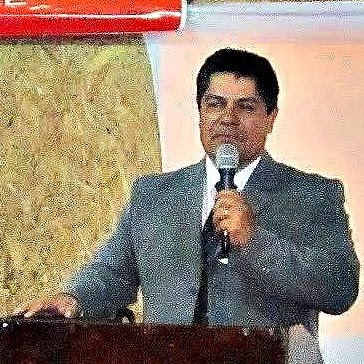The image depicts a pixelated scene of a middle-aged man, possibly Hispanic or Caucasian, speaking at a podium. He has short black hair and is dressed in a dark charcoal gray suit jacket, paired with a black tie and a white collared shirt. His expression is stern, with his mouth turned downward in a scowl. In his left hand, he firmly holds a black microphone with a silver top, while his right hand rests on a dark brown podium, which reaches up to his chest. The background is notably blurred, with the left side featuring a brownish, stone-like texture and the right side dominated by a pink hue. Additionally, in the upper left corner, there is a strip of bright red with white stripes, although its details remain indiscernible due to the image's pixelation.